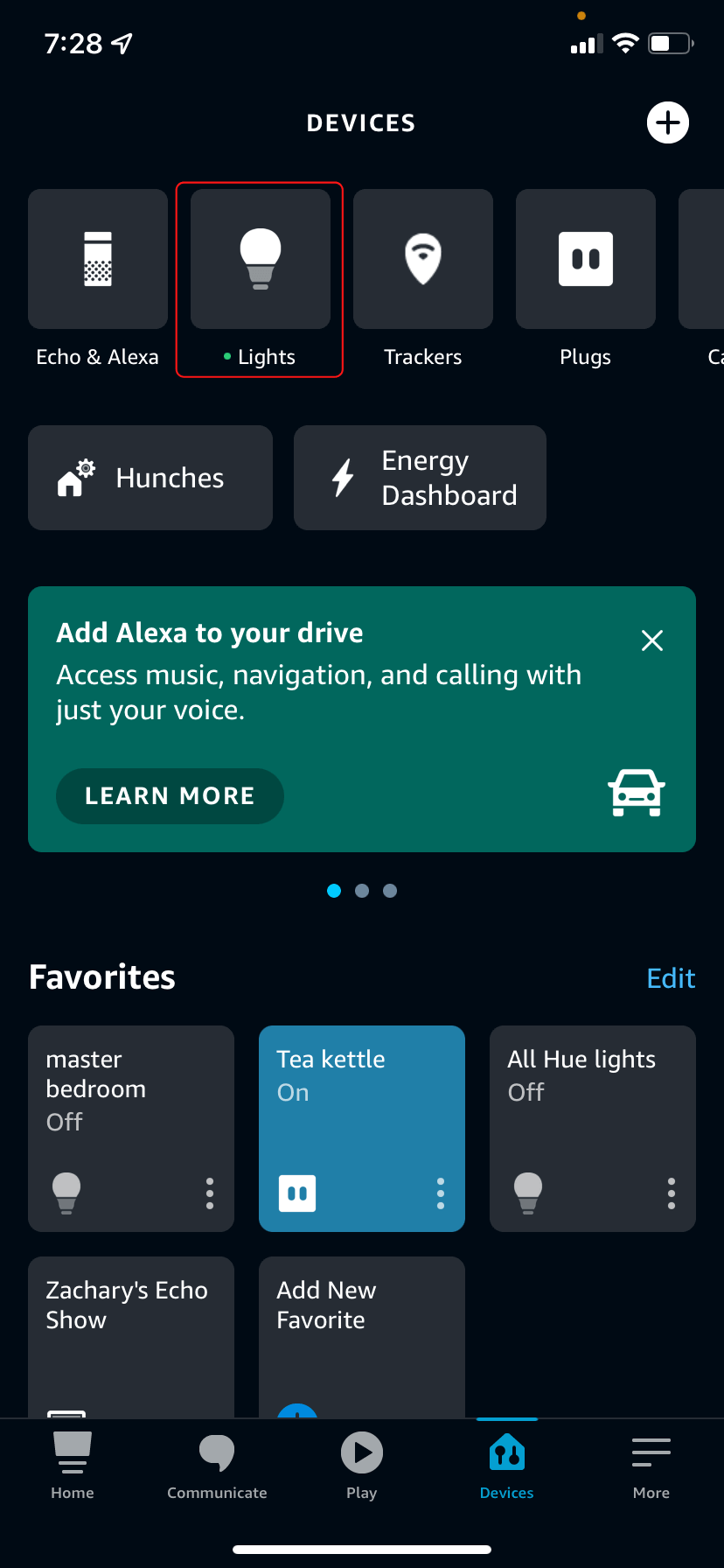Screenshot of a smartphone displaying a home automation control dashboard. The background is black with a status bar at the top. In the top left corner, the time reads 7:28. To the right, an upward-pointing arrow icon is visible. On the right side of the status bar, there's a battery icon with a gray border and a half-filled white battery level. Next to it, a full Wi-Fi icon and a four-bar internet signal indicator, with three bars in white and one in gray.

Below the status bar, the word "DEVICES" is written in all capital white letters. To the right, there's a white circle with a black 'X' inside it. Beneath this circle, there's a square containing the Alexa icon, and below it, "Echo and Alexa" is written in white. 

Next, there is a light bulb icon inside a gray square marked with "Lights" in white text, bordered by a red square. Following that, there are icons for "Trackers" and "Plugs."

Further down, a tab labeled "Hunches" with a home icon to its left is present, followed by a "Energy Dashboard" tab featuring a light bulb and a voltage icon. Below these tabs is a large teal rectangle with the text "Add Alexa to your Drive," a small 'X' on the right side, a car icon at the bottom left, and two horizontal lines to the left of a dark green and white tab labeled "Learn More." 

Centered below is a navigation dot indicator with a blue dot followed by two gray dots. To the left, the word "Favorites" is in white, and to the right, "Edit" is in white. There are three control icons across the screen, with the outer two in gray and the middle one in blue. Below these, there are two more control icons.

At the bottom, a black border contains navigational options in gray: "Home" with a home icon, "Communicate" with a talk icon, "Play" with a play icon, "Devices" in blue with a home-like icon, and "More" with a gray icon.